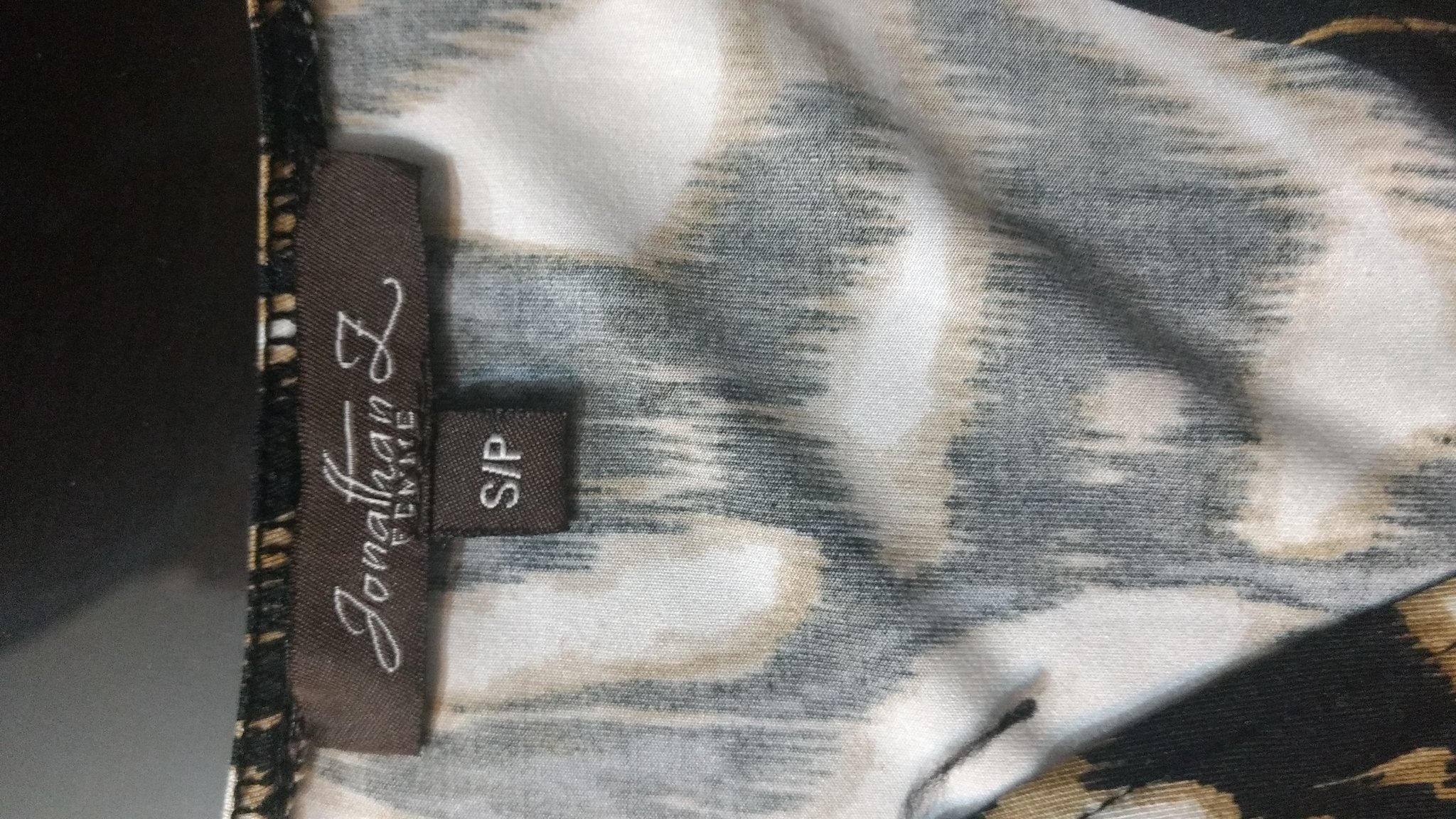This digital photograph captures the inside of a women's shirt, displayed somewhat sideways. The shirt predominantly features a mix of white, light brown, and black colors with various spots throughout the fabric. The colors on the inside are notably less vibrant compared to those on the outside. The shirt appears to be black with some tan spotting on the outer part and is primarily light with visible prints from the inside.

In the bottom right corner, a rectangular black tag is attached, facing right and displaying the name "Jonathan L" in cursive, accompanied by a faint text beneath it. Alongside this tag is a smaller square tag indicating the size "S/P" in white font. The shirt's stitching, which can be seen near the top of the image, is black.